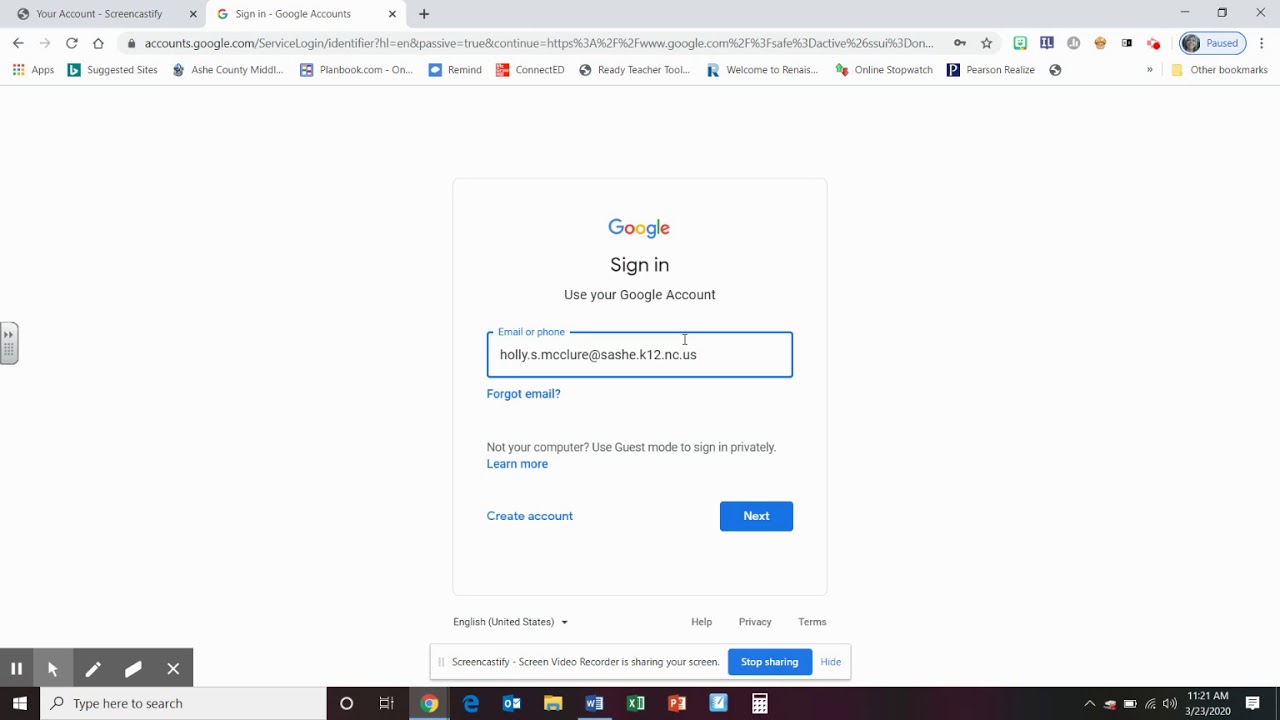A detailed screenshot of a Google sign-in page displayed on a computer screen. The background is predominantly white. At the very top of the screen, a gray horizontal bar spans the entire width. The first tab in the gray bar contains black text reading "Your Account Screencastify." Adjacent to it is a white tab featuring the Google emblem, followed by another tab titled "Sign In Google Accounts."

Below this bar is the search bar displaying "accounts.google.com," along with various icons indicating a paused state. Listed below the navigation tabs are a series of bookmarks: "Apps," "Suggested Sites," "Ash County Minute," "planbook.com," "Remind," "ConnectED," "ReadyTeacherTool," "Welcome to Rene's," "Online Stopwatch," "Pearson Realize," and "Other Bookmarks" positioned furthest to the right.

Centered on the screen is a prominent sign-in box. At the top of the box sits the Google emblem, followed by black text reading "Sign In." Below this, the instruction "Use Your Google Account" is prominently displayed. The prompt "Email or Phone" appears next, with a text box underneath showing the pre-filled email address "holly.s.mcclure@sashay.k12.nc.us." Under the email field, a blue hyperlink titled "Forgot Email?" can be seen, followed by "Not Your Computer? Use Guest Mode to Sign In Privately," and another link titled "Learn More." On the right side of the sign-in box, a blue rectangle with white text saying "Next" is displayed.